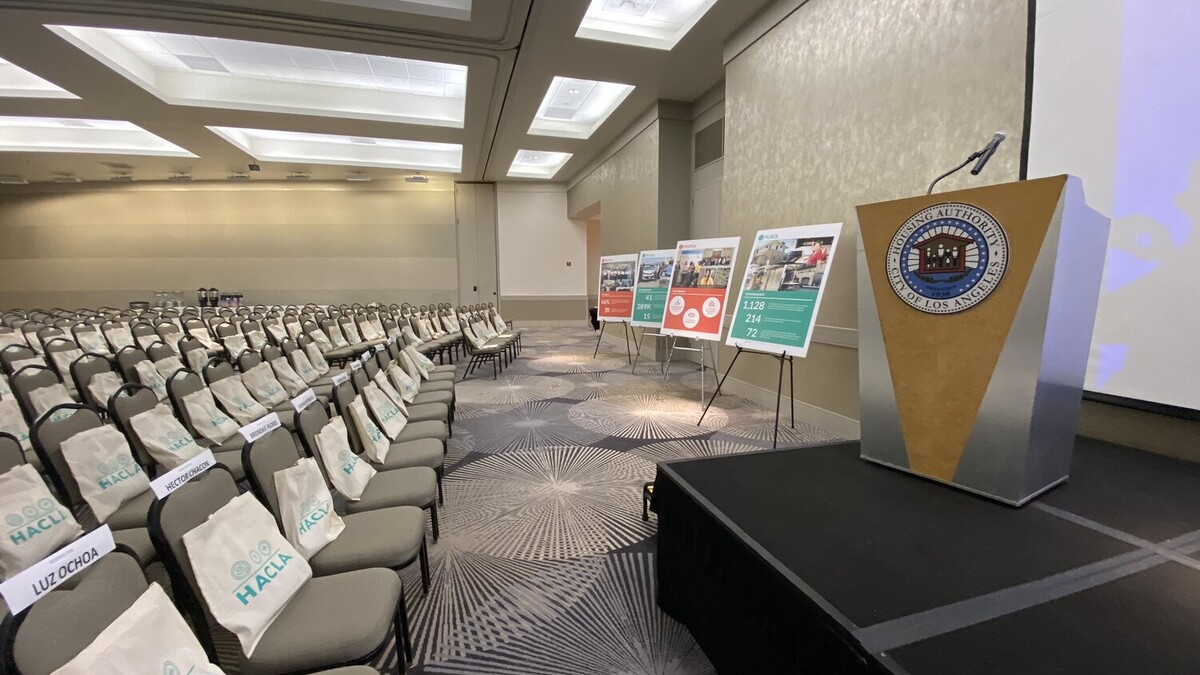This image captures a detailed view of a spacious conference room, likely set up for a forthcoming event. The large room is equipped with at least a hundred seats arranged neatly towards the back and both sides of the space. Central to the scene is a small black stage positioned on the right side, furnished with a podium bearing the logo of the City of Los Angeles. A microphone is attached to the podium for speakers.

On the left side of the room, several boards on stands present various texts and images, appearing to be instructional or informative materials for attendees. The overall aesthetic of the room is neutral, dominated by beige tones, with minimal color except for the boards. The floor features subtle circular designs, adding a modest decorative touch without overwhelming the space.

Each seat in the room holds a white paper bag labeled "H-A-C-L-A," likely containing materials or gifts for the conference participants. In the second rows, the seats are marked with labels denoting specific attendees, with identifiers such as "L-U-Z-O-C-H-O-A" rather than personal names. These markers are probably known to the attendees. The room exudes a calm and organized atmosphere, suggesting careful preparation for an educational or professional gathering.